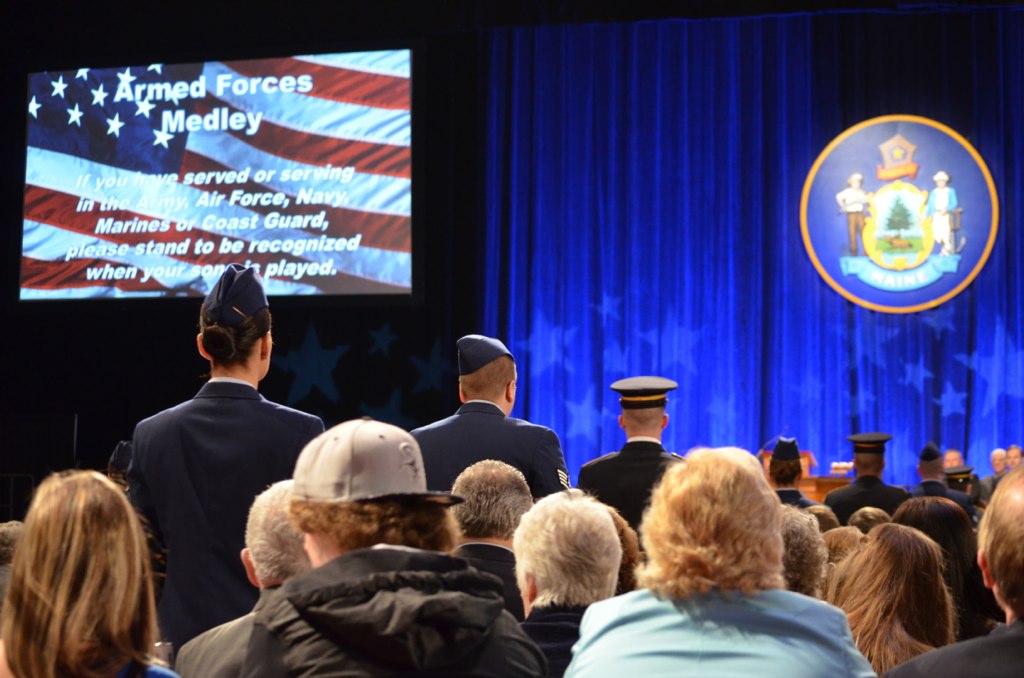In this detailed image from a military presentation, we observe a group of audience members. They appear to be seated, with men and women alike visible from the back. An aisle runs to the left side of these seated individuals, down which two men and a woman, all in military uniforms, are walking. The two men in front are wearing either thin black or blue hats; one of these hats, possibly worn by the leading man, has a flat top resembling a captain's hat. They proceed towards a stage adorned with a drawn blue curtain that emits lights resembling stars. To the left of this curtain, a screen reads: "Armed Forces Medley. If you have served or are serving in the Army, Air Force, Navy, Marines, or Coast Guard, please stand to be recognized when your song is played." An American flag subtly forms the backdrop of the screen. Additionally, there is mention of a seal on the curtain, featuring two figures around a central tree-like emblem.